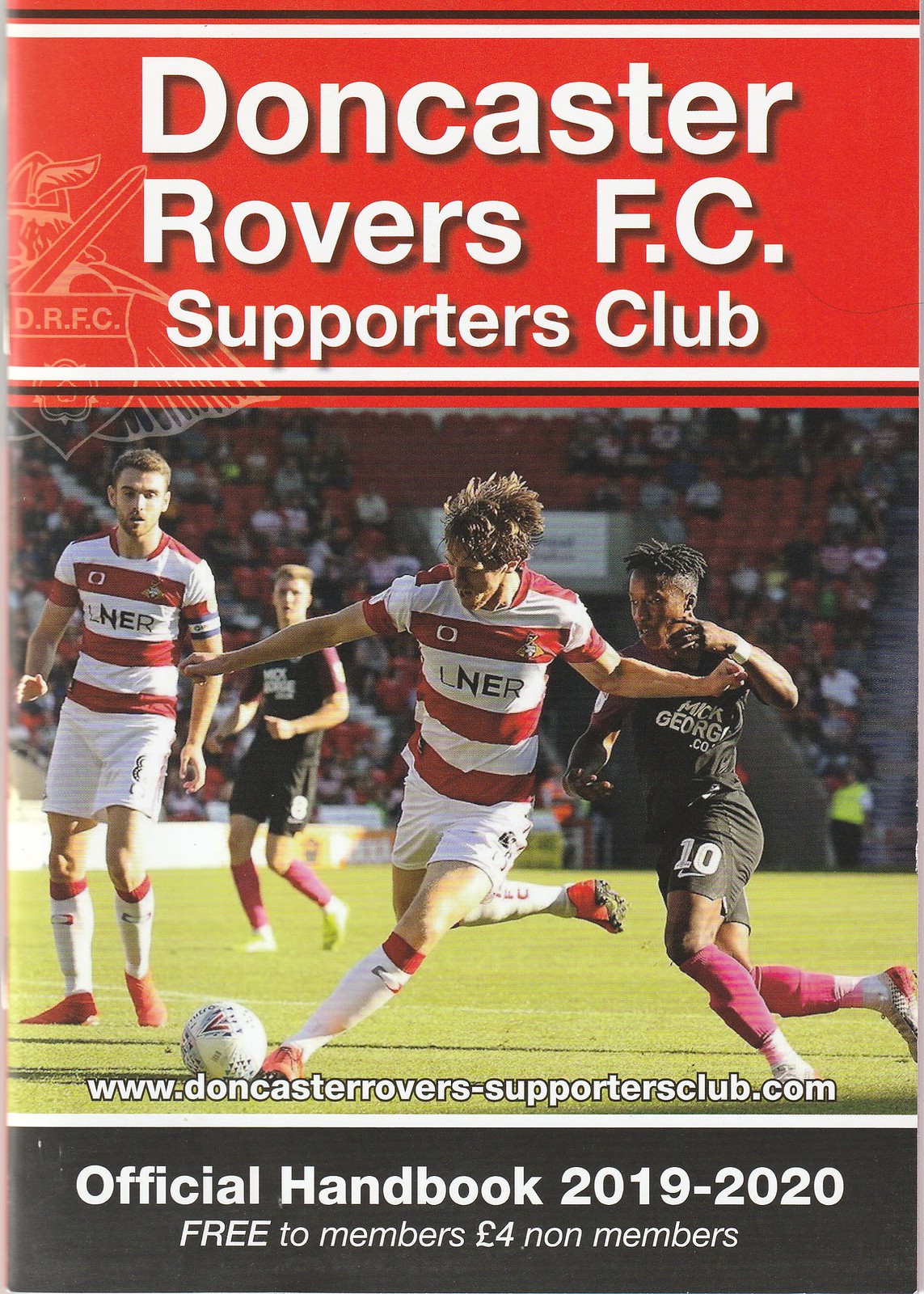The image depicts the cover of the Doncaster Rovers F.C. Supporters Club 2019-2020 Official Handbook. The top third of the cover features a red background bordered by white and black lines. Centered in the red section are the words "Doncaster Rovers F.C. Supporters Club" in white font with black shadowing, alongside a partial logo of a Viking carrying a shield with the letters D.R.F.C. in off-white outline on the left side.

Beneath this, the main image showcases a live soccer game with four players on a green field. The center of the action features a player with olive skin, dark hair, wearing a red and white striped jersey with 'LNER' on the chest, white shorts, white socks, and red cleats, attempting to kick a white soccer ball with his right foot. Right beside him is an African-American player with short braided hair in a black jersey, number 10, maroon socks, and white and red cleats seemingly trying to block the kick. On the left side, there are two more players observing the game: one is a Caucasian male with short dark hair, in a red and white striped jersey with 'LNER' on the chest, white shorts, white socks, and red cleats. The other is a young Caucasian male with blonde hair, wearing a black jersey, black shorts, maroon socks, and white cleats. A large crowd can be seen in the background, with red seats visible where the crowd thins.

At the bottom of the image, a website "www.doncasterrovers-supportersclub.com" appears in white font. The final section of the cover has a charcoal gray background with the text "Official Handbook 2019-2020, Free to Members, Four Pounds Non-Members" written in white font.